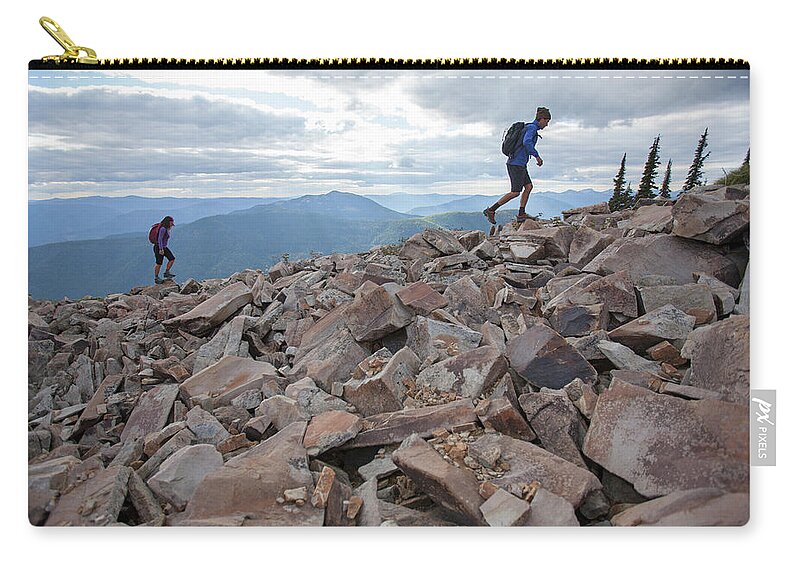The image features a black rectangular pouch with a golden zipper running along its upper edge. Stitched onto the side of the pouch is a detailed photo of two hikers ascending a rugged, rocky hill composed of large, jagged stones in shades of gray and red. In the foreground, a woman wearing black shorts, a long-sleeved purple shirt, hiking shoes, a red backpack, and sporting brown hair is positioned at a lower level. Ahead of her is a man, dressed in a blue jacket and black shorts, with orange and gray (or possibly red and gray) hiking shoes. Both individuals carry camping equipment. The background of the photo reveals a lush mountain range with grassy slopes under a sky filled with many gray clouds. In the upper right of the background, distant trees can be seen. To the lower right corner of the image, a logo reading 'PXPixels' is visible. The entire scene is beautifully depicted against a white background, enhancing the product's features and the adventurous spirit captured in the image.